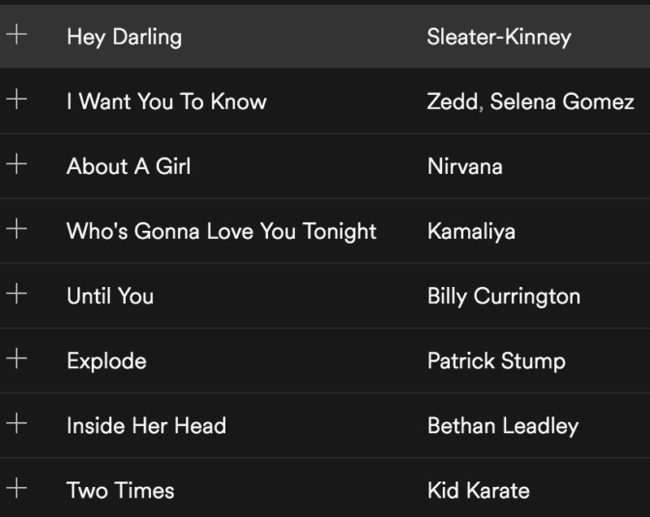Here is the cleaned up and descriptive caption:

---

The image displays a sleek tablet screen showcasing a music playlist. The interface features a minimalist design with a black background and white lettering. Each song title on the list is accompanied by a plus sign, presumably for expanding the selection with additional options. The playlist includes the following tracks:

1. "Hey, Darling" by Sleater-Kinney
2. "I Want You to Know" by Zedd and Selena Gomez
3. "About a Girl" by Nirvana
4. "Who's Gonna Love You Tonight" by Camellia
5. "Until You" by Billy Currington
6. "Explode" by Patrick Stump
7. "Inside Her Head" by Bethan Leadley
8. "Two Times" by Kid Karate

Notably, the presence of artist Kid Karate and the revelation of Selena Gomez's involvement in music may come as a surprise to some viewers. The interface offers no additional settings or pages – it is simply a straightforward playlist ready to be played.

---

This caption provides a clear and detailed description of what is displayed on the tablet screen, covering the song titles, artists, and overall interface.